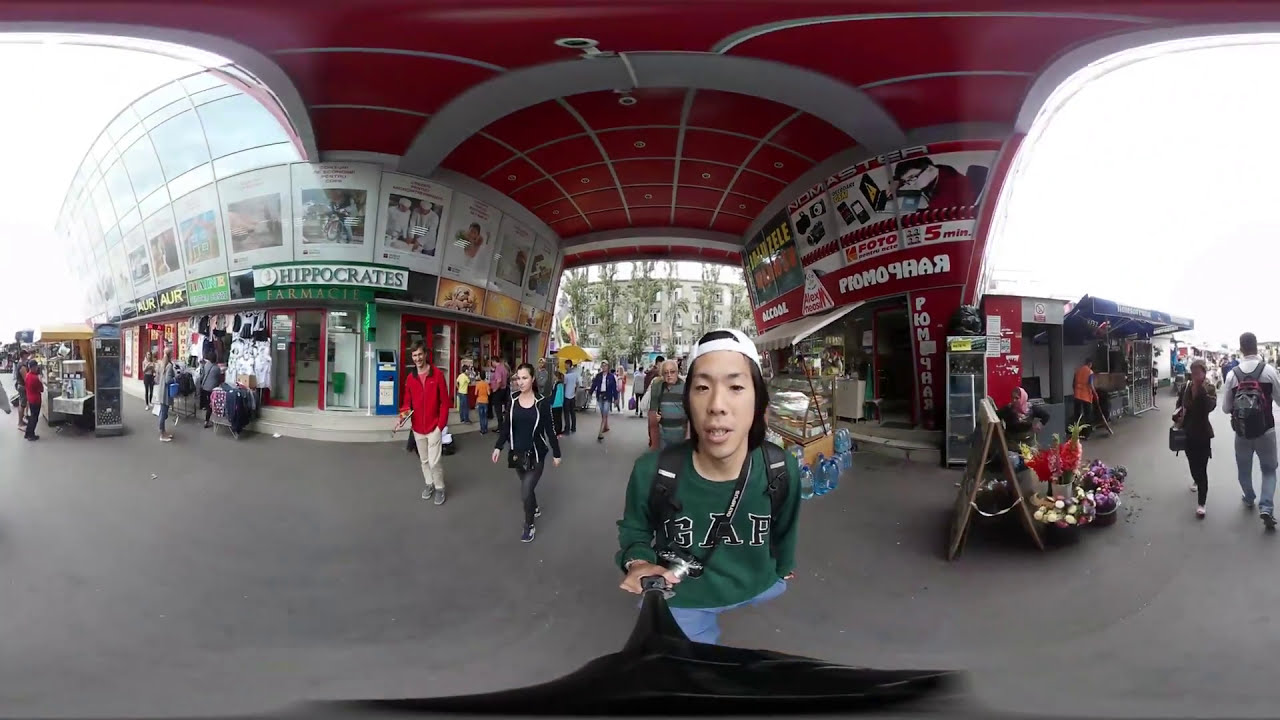In this panoramic, color photograph, a young Asian man stands at the center, capturing a selfie with a selfie stick. He wears a white baseball cap turned backwards, a dark green GAP sweatshirt, and blue jeans. His black hair falls to his shoulders, and a black strap from a silver camera hangs around his waist while backpack straps are visible on his shoulders. He holds the selfie stick in one hand, with the other hand tucked in his pocket.

The backdrop reveals a bustling outdoor shopping street with vendor kiosks and numerous pedestrians engaging with the displays. Overhead stretches a dark red arched roof structure, partially open to reveal an overcast, gray sky. On the left, a sign reads "Hippocrates" on a green background, while on the right, a sign is present but unreadable, obscured by a person. The scene is set against a landscape-oriented panorama, accentuating the lively atmosphere of the shopping district.